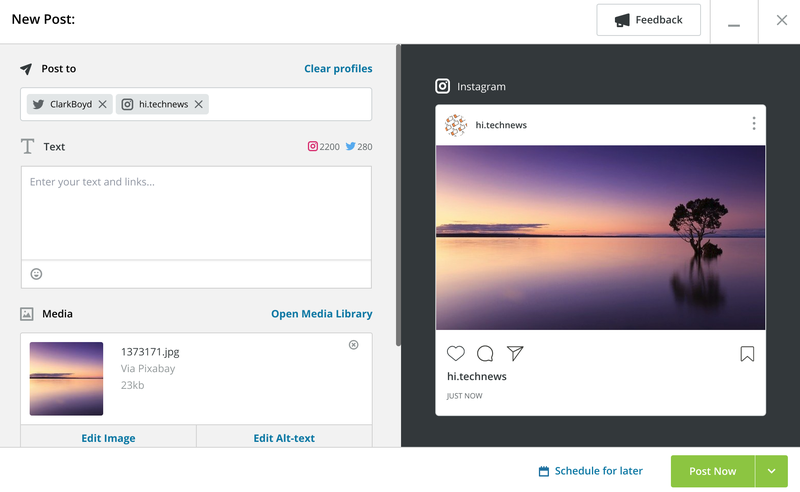### Instagram Post Screenshot Description

The screenshot captures both the composition process and the final Instagram post. 

#### On the Right:

- **Post View**:
  - **Border & Header**: The image is framed by a black border with the Instagram logo at the top.
  - **Image**: The post features a serene evening seascape, likely of a lake. The sky is a gradient of purple hues, darkening towards the right. The lighter area at the bottom left suggests the sun is setting, casting its glow across the water's surface. A single tree emerges from the water on the right, its reflection mirroring its form in the still lake.
  - **Username & Timestamp**: Below the image, the username "@hi.technews" is visible along with the timestamp indicating it was posted 'just now'.

#### On the Left:

- **Creation Interface**:
  - **Header**: A grey box labeled "New Post" sits at the top left, indicating the stage of the posting process.
  - **Post Details**: 
    - **Destination**: The post is being shared to both Twitter and Instagram.
    - **Text Box**: An empty text field is provided for adding a caption or description, though none has been entered yet.
  - **Media Details**:
    - The image file is listed as "137371.jpg," with a size of 23 kilobytes.
  - **Options**: Two buttons allow the user to edit the image or its alt text, highlighted in blue on the grey background.
- **Action Buttons**:
  - **Post Timing**: At the bottom right, the interface options to "Post Now" in a green box or "Schedule for Later."

This Instagram post captures the tranquility of nature at dusk, skillfully blending technology with natural beauty in a purple sky and reflective waterscape.